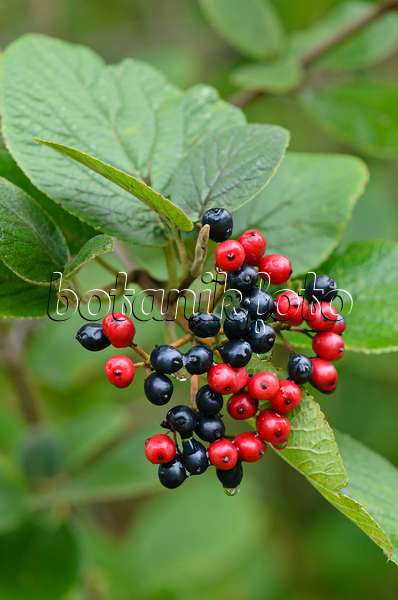This photograph, likely from the company "Botanic Photo" (as indicated by the watermark that partially spans across the berries and leaves), features a detailed close-up of a cluster of small red and dark blue (or black) berries set against a background of large green leaves. The precise organization of the berries shows a mix of color with the red berries predominantly on the right and the blue/black berries primarily on the left, though they intermingle in various patterns. There are approximately 30 berries in total, with the configuration including specific groupings such as one black berry beside two red berries, followed by a swirl of nine blue berries, a trio of red berries, a solitary black berry, an L-shaped cluster of six red berries with a black one above, and a final mix featuring ten red berries surrounded by seven black ones, plus one red berry off to the side. The green leaves, some flipped to reveal their lighter undersides, form a rich and textured background, although they are blurred to keep the focus firmly on the colorful berry cluster upfront.